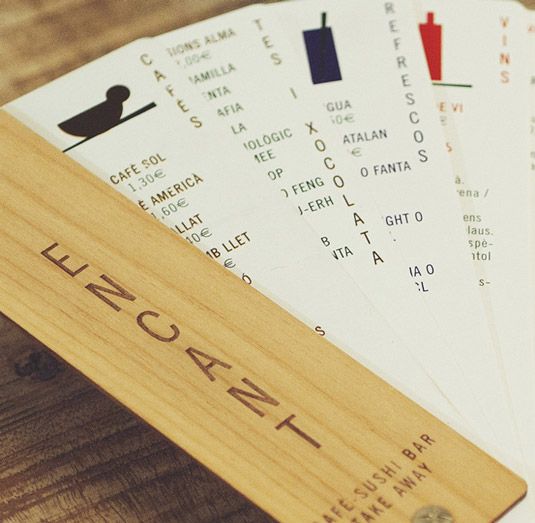This square photograph captures a wooden table with a detailed texture, prominently positioned in the middle of the image. On the table lies a fan-shaped wooden object, possibly a menu, labeled "Encant Cafe Sushi Bar Takeaway" in vertical writing along its handle. Below this primary text, additional horizontal lettering appears, though it is not entirely legible. Fanning out from a rivet or screw at the bottom, there are six sections that resemble cards or menu sheets. Each section appears to display menu items and prices, with visible words such as "Cafe Sol," "America," "Cafes," "Tess," "Xocolata," and "Refrescos." The cards, adorned with small images like a bird or a soda drink, are unfortunately not fully extended, making some text difficult to read. The scene is likely set indoors, with the arrangement suggesting a possible restaurant setting, given the combination of the fan-shaped menu and the café-themed text. The color palette consists of various shades of brown, white, black, and red.